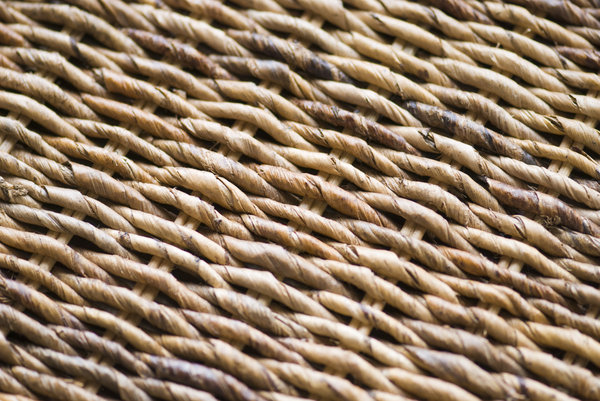This detailed close-up image captures the intricacies of a woven basket made from natural fibers. The material appears to be a tightly woven wicker, showcasing a pattern of twisted, cylindrical pieces interwoven in an over-and-under fashion. Dominated by light tan hues, the basket also features patches of darker browns and subtle grayish stains, adding a natural variation to the texture. The weave is exceptionally precise, with some strands slightly thicker than others, and the ribbing elements are visible through the tiny gaps. The basket leans diagonally toward the upper right corner, and the image, free of text or other distractions, presents an authentic, unaltered view of the craftsmanship.